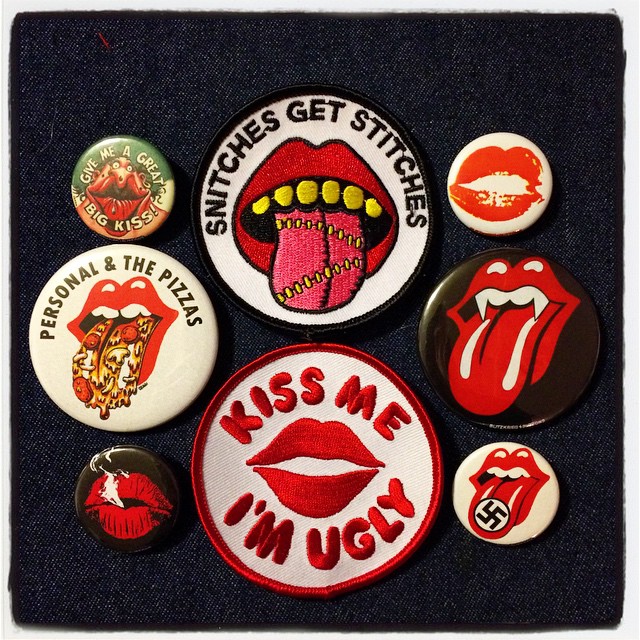This image displays a collection of eight buttons and patches on a black fabric backdrop, with a common theme of lips or mouths. The items are arranged in a staggered fashion:

1. **Top Left**: A small button features the phrase "Give a great big kiss" accompanied by a picture of a slightly yucky, or disgusted, face.
   
2. **Next Item Down**: A fabric patch with the text "Snitches get stitches," depicts a mouth with yellow teeth and a tongue that has stitches on it.

3. **Next in the Row**: Another button with white as its base color simply shows red lips, a classic Rolling Stones logo.

4. **Following Item**: A white button features the text "Personal and the pizzas," showcasing a mouth with a tongue extended and pizza sauce on it.

5. **Next in Line**: A fabric patch with a circular white stitching says "Kiss me, I'm ugly" alongside big red lips.

6. **Bottom Row**: A black button portrays red lips with smoke coming out.

7. **Bottom Left**: A black button showing red lips with white teeth and a long tongue hanging out.

8. **Bottom Right**: A white button with a red mouth and tongue illustrated with controversial imagery including swastikas.

The collected items bear common details like red lips, tongues, and provocative phrases, illustrating a blend of rock band iconography, such as the Rolling Stones' lip logo, and edgy, rebellious expressions.